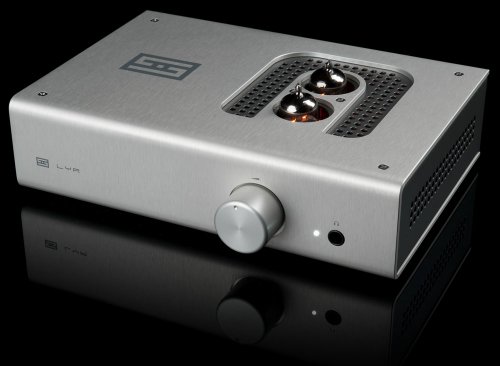The image features a small, flat, rectangular silver electronic device that appears to be a piece of audio equipment. The front is adorned with a large, silver adjustment knob that has a dot indicator. The right half of the device's face has a screen-like top section, housing two silver buttons. Additionally, a small black dot is in the right corner, resembling an LED light. There's a black headphone jack located on the bottom right, identified by a headphone logo above it.

A unique feature includes a U-shaped metal grating on its side and the device boasts a logo of two interconnected S's with a dot in the middle. Overall, this device has a brushed metal finish, giving it a blend of modern and slightly retro aesthetics. The entire setup sits on a black reflective surface, enhancing its sleek, futuristic appeal.